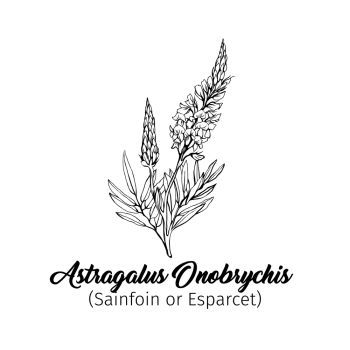The image is a detailed black and white hand-drawn illustration of a plant, depicting the Astragalus onobrychis. The drawing features a central stem with four branches. The two lower branches are adorned with multiple thin leaves, giving a delicate, feathery appearance. The upper branches display two distinct flowers: the left flower is thinner and conical, resembling a wheat germ or tall grass, while the right flower is larger with more pronounced petals. The hand-drawn texture suggests the use of pencil or ink. Below the illustration, the plant's Latin name, "Astragalus onobrychis," is written in bold black cursive. Beneath this, in regular black font within parentheses, the common names "Sainfoin" or "Esparcet" are provided, clarifying the plant's genus and classification. The background is plain white, ensuring the focus remains on the detailed botanical artwork.